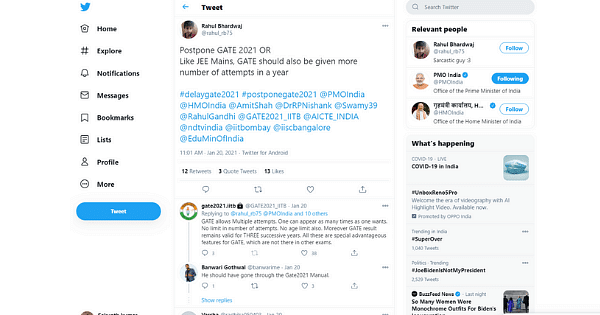This image appears to be a screenshot of a computer screen displaying a Twitter page, characterized by a white background. The top-left corner features Twitter's iconic blue bird logo. Directly beneath the logo is a vertical array of eight icons in black, including Home, Explore, Notifications, Messages, Bookmarks, Lists, Profile, and More. Below these icons, there is a blue, rounded rectangle with the white text "Tweet."

In the central section of the screen is a Tweet authored by Rahel Bardra. At the top of this Tweet section, 'Tweet' is displayed in bold with a blue arrow to the left. Rahel Bardra's Tweet content follows, and beneath the main Tweet, various hashtags and shoutouts appear in blue. The Tweet has garnered 12 retweets and 13 likes, and it was posted at 11:01 AM on January 20th, 2021. Below this main Tweet are a series of additional Tweets not fully described in the caption provided.

On the right-hand side of the screen is a grey rectangular sidebar. At the top of this sidebar are darker grey letters followed by a section titled "Relevant People" in bold black font. The first relevant person is Rahel Bardrage, whose icon features a man's face with predominantly brown and white colorations. The next item is a profile for 'P-I-B-O, India,' accompanied by an icon of a man from the shoulders up, wearing something orange and appearing to either have white hair or be bald.

Further down the sidebar, under the section "What's happening," you can find updates about COVID-19 in India, alongside other pieces of information that extend towards the bottom of the screen. While the primary background of the page is white, the text boxes located in the bottom right-hand corner of the image have a light grey coloration.